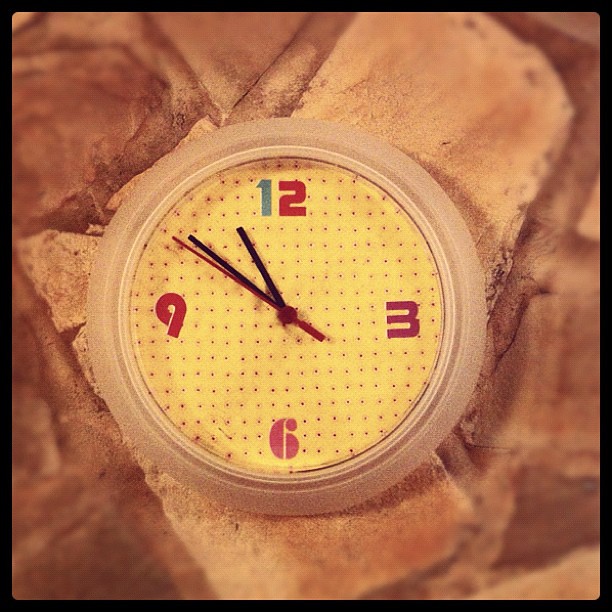The image features a round clock face with a natural wood finish frame, centrally placed on a brown and tan stone surface with an orange hue, possibly a floor, wall, or mantelpiece. The stone area is bordered by a dark black line that outlines the entire image. The clock face itself is yellow and patterned with small brown dots arranged in rows, giving it a graph paper-like appearance. Only the 12, 3, 6, and 9 are present among the numbers, with a distinctive feature: the digit '1' in '12' is blue, while '2' in '12,' along with the '3,' '6,' and '9' are red. The clock has three hands – an hour hand and a minute hand, both black, and a second hand, which is red. The bezel surrounding the clock face is a thick off-white or translucent white, creating a striking contrast against the detailed textured stone background.